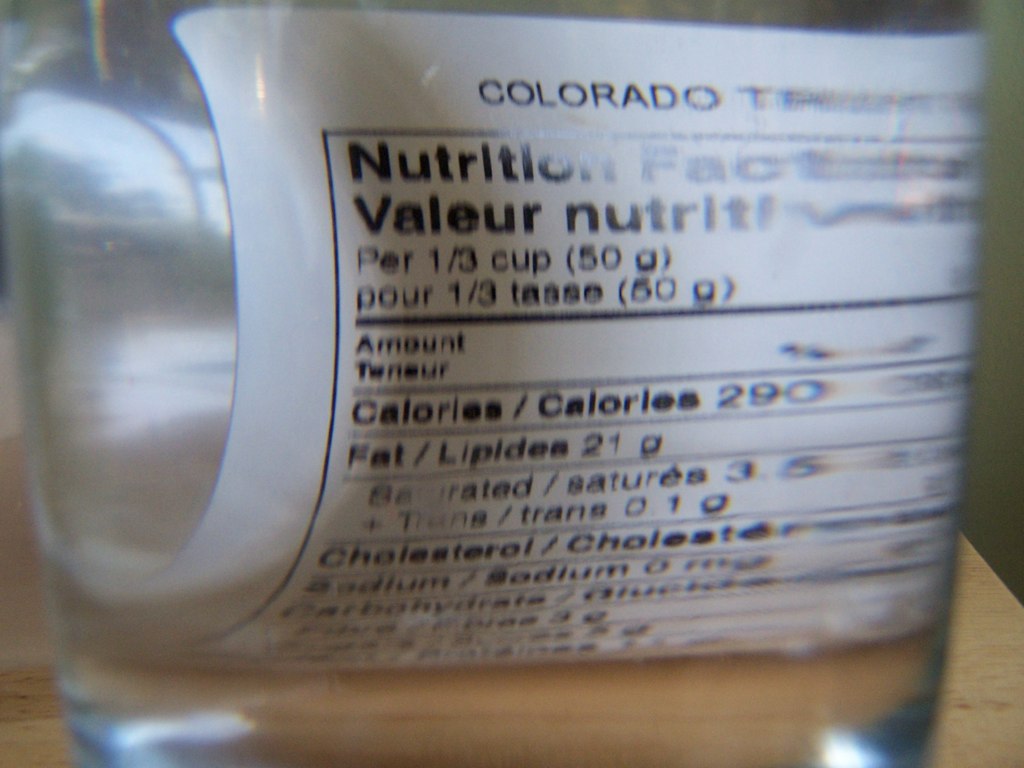The image depicts a nutrition facts label written in what appears to be Portuguese, detailing the nutritional value of an unidentified liquid product. The label, though slightly distorted and blurry, includes information such as serving size, calorie count, fat content, cholesterol, sodium, and carbohydrates, each listed with their corresponding amounts. There is also a mention of Colorado, but the context is unclear due to the image's poor quality. Overall, the label is difficult to read clearly, making it challenging to identify the product specifically.